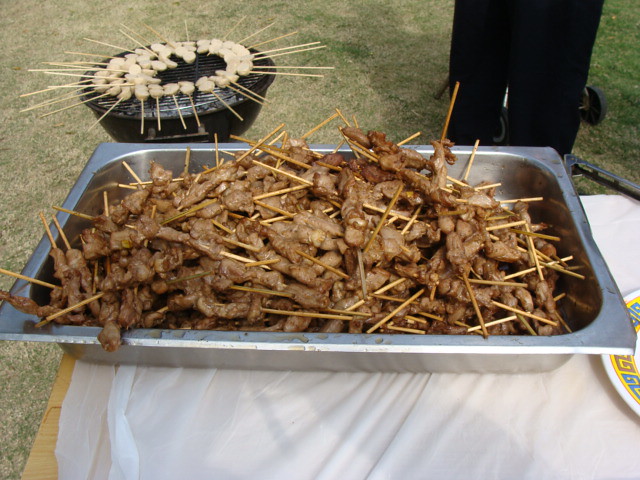In the photo, a picnic scene is depicted with a white plastic-covered wooden table set outdoors on a green lawn, some patches of which are a lighter brown. Dominating the table is a large, deep, rectangular metal pan brimming with wooden skewers of grilled meat. These meat skewers, possibly chicken or pork, have a browned, almost grayish appearance with some burnt spots and are piled high, even past the lip of the pan. To the right of the pan sits a distinctive white plate adorned with a yellow band and a blue and red abstract, Greek-like pattern around its edge.

In the background, a black, half-cylinder charcoal grill with handles is filled to capacity with skewers of pale, uncooked scallops, indicating they are still in the process of cooking over hot coals. The entire scene suggests the setup might be for a large outdoor gathering or a street vendor-inspired event. Additionally, a black, wheeled trash can is visible beside the table, adding to the casual outdoor vibe of the barbecue.